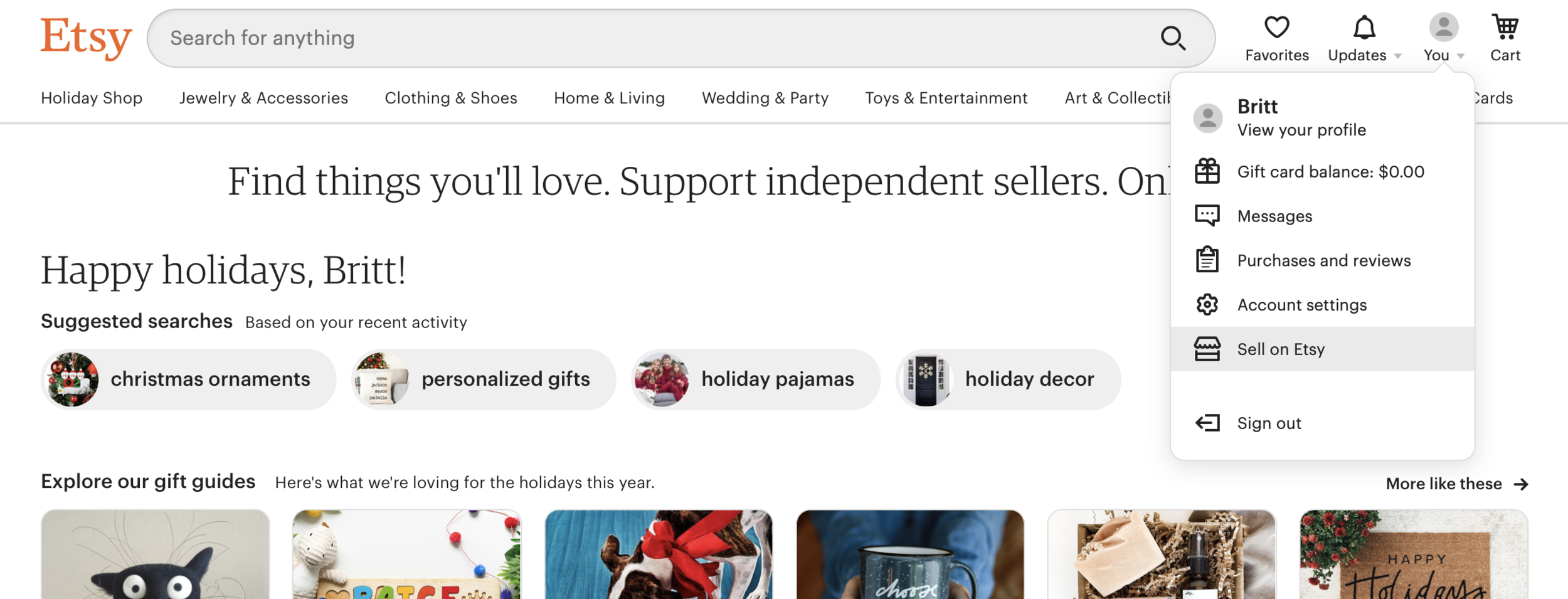A screenshot of an Etsy webpage is shown with the primary navigation and user options clearly visible. At the top, there is an orange bar with the text "EMTSYXZ." Below it, there is a gray oval shaped search bar that contains the words "Search for anything" alongside a black magnifying glass icon. To the right, a heart icon with "Favorites" and a bell icon with "Updates" are displayed. Additionally, there is a gray circle featuring an outline of a person with the word "You" in black text, a shopping cart icon labeled "Cart," and an item count inside the cart.

A user has clicked on the "You" section, triggering a white pop-up menu. The menu lists options in black text: "Brit," with "View your profile" below it, "Gift card balance: $0.00," "Messages," "Purchases and reviews," "Account settings," and a highlighted option "Sell on Etsy." The "Sign out" option appears at the bottom of this menu.

On the left side of the screen, a vertical black menu features categories: "Holiday Shop," "Jewelry & Accessories," "Clothing & Shoes," "Home & Living," "Wedding & Party," "Toys & Entertainment," and partially visible "Collectibles." The list is interrupted by the pop-up menu.

Beneath the categories, a message partly obscured by the pop-up reads: "Find things you love, support independent sellers, on..." further cut off by the pop-up. Additional text on the page greets the user with "Happy holidays, Brit" and "Suggested searches based on your recent activity" with items such as "Christmas ornament," "Personalized gift," "Holiday pajamas," and "Holiday decor" listed. The page also mentions "Explore our gift guides," "Here's what you're loving," and "Here's what we're loving for the holidays this year." To the far right, it says "More like these."